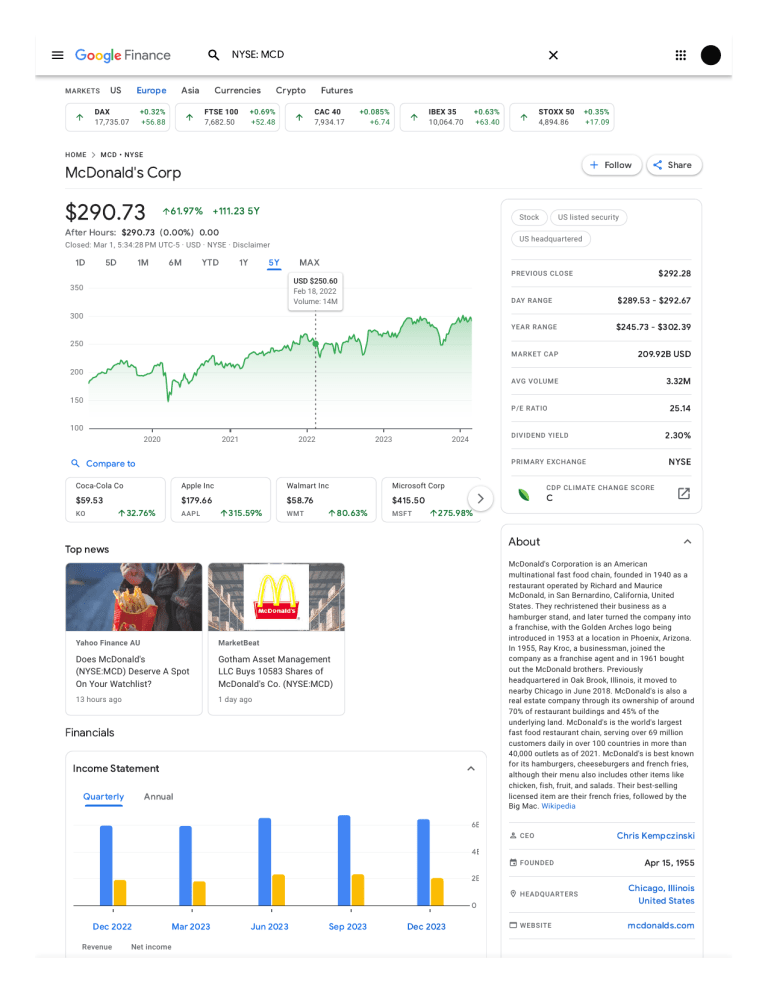A screenshot of the Google Finance interface is displayed. In the top left corner, the recognizable Google Finance logo is prominently featured. Adjacent to the logo is a search bar, which shows an active search for "New York Stock Exchange MCD," referring to McDonald's share price. 

Spanning across the top of the screen are panels providing an overview of several common indices, including the DAX, the FTSE 100, the CAC 40, the IBEX 35, and the STOXX 50. Above these panels, there are navigation tabs for selecting different market sectors, namely US, Europe, Asia, currencies, crypto, and futures.

The main section of the screen is dominated by a detailed chart displaying the McDonald's share price, currently marked at $290.73. The chart is set to a five-year timescale, illustrating the fluctuations in McDonald’s share price over that period. The chart setting options allow for timeframes ranging from one day to the maximum available span, although the specific extent of the 'max' option is unclear.

To the right of the chart, a sidebar presents key metrics, including the previous close price, the day range, the price variation over the last day, the year range, market capitalization, and average trading volume. Further down, additional panels provide general information about McDonald's, recent news updates, and income statements. These details offer a comprehensive overview of the McDonald's Corporation, enriching the user's understanding of the company's financial status and market position.